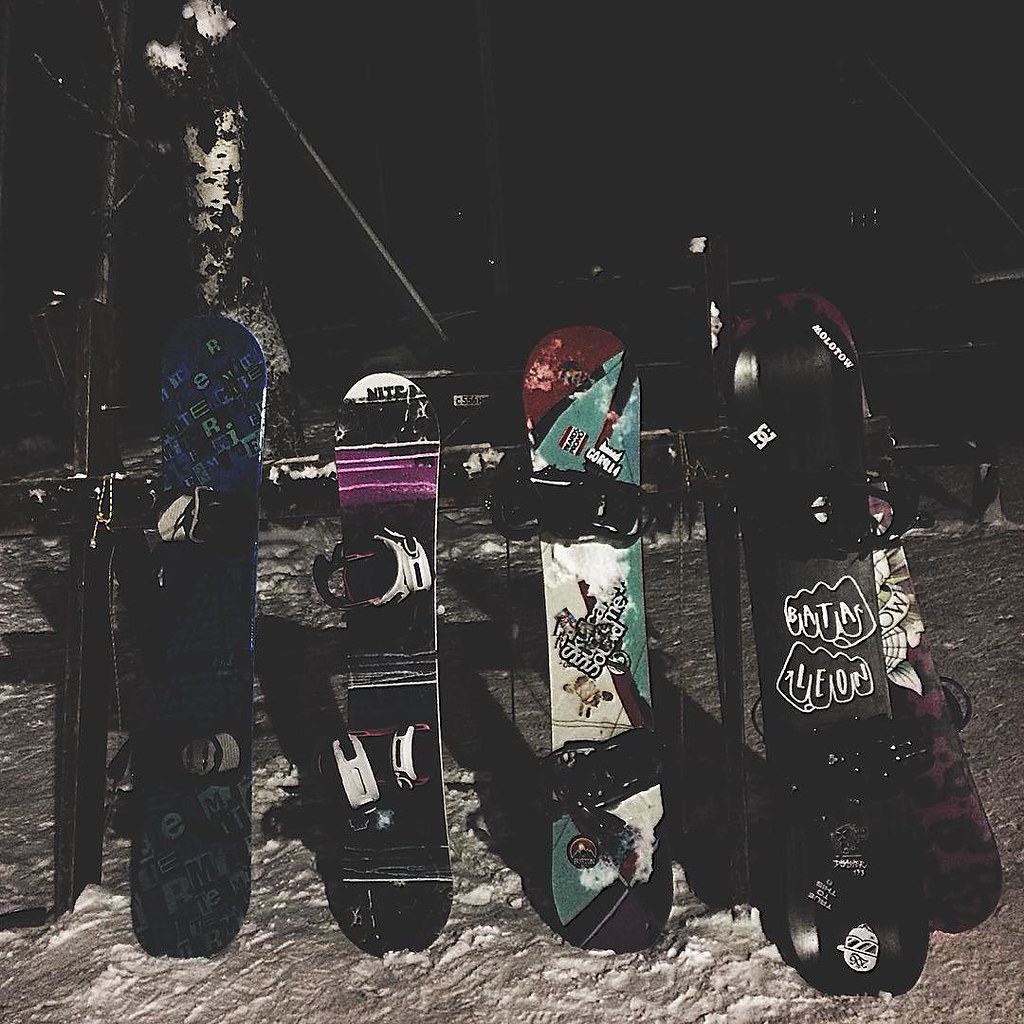The photograph captures five snowboards stacked up against a black fence on a well-packed snowy hill at night. Illuminated by a significant flash or light, the image reveals shadows cast by the boards against the white snow, emphasizing the night's darkness. 

From left to right, the first snowboard is blue with green and black writing, though the text is too small to read. The second snowboard, shorter than the first, is black with three white stripes and a pink splotch at the top, ending in a white tip. The third snowboard is slightly longer, black and teal with unreadable writing in the middle and a red tip. The fourth snowboard is solid black, featuring the simple outline designs of two fists, one above the other. The knuckles of the top fist spell "B-A-T-A," while the bottom fist reads "L-E-O-N." This board partially obscures the fifth snowboard, which appears to be a reddish-black color.

Behind the boards stands a beech or birch tree, tied up presumably due to stability issues. The nighttime setting and the lighting conditions create a dramatic effect, with the snowboards and the tree prominently standing out against the dark background.